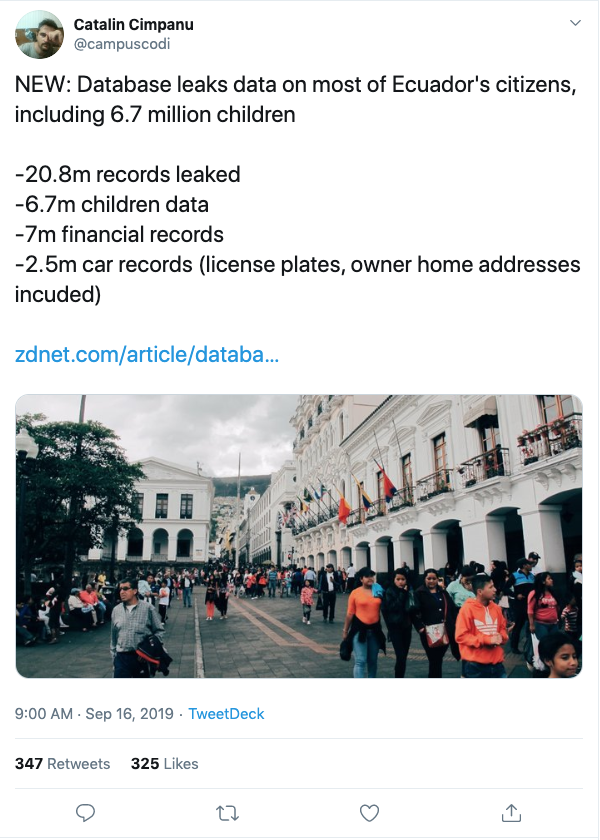Here is an improved and detailed caption based on the provided voice description:

---

**Screenshot from Twitter:**

The display image features a man with short brown hair, wearing a gray t-shirt. His name appears as "Catalin Cimpanu" and is followed by the handle "@CampusCodi."

A tweet in bold reads:

**New:** "Database leaks data on most of Ecuador's citizens, including 6.7 million children."

A bulleted list follows:

- **20.8 million records leaked**
- **6.7 million children's data**
- **17 million financial records**
- **2.5 million car records (including license plates and owner's home addresses)**

A link to the detailed article is provided: "zdnet.com/article/data..."

Beneath the tweet is an image depicting a protest scene. Several people are marching outside two white, old-fashioned buildings under a gray sky. The surroundings feature green leafy trees and a cobblestone road. Many protesters are wearing orange and black shirts. Political flags are visible, suggesting a demonstration in front of a government building. In the background, a hint of a mountain terrain can be seen.

---

This caption offers a clear and detailed description of the Twitter screenshot and the accompanying image.